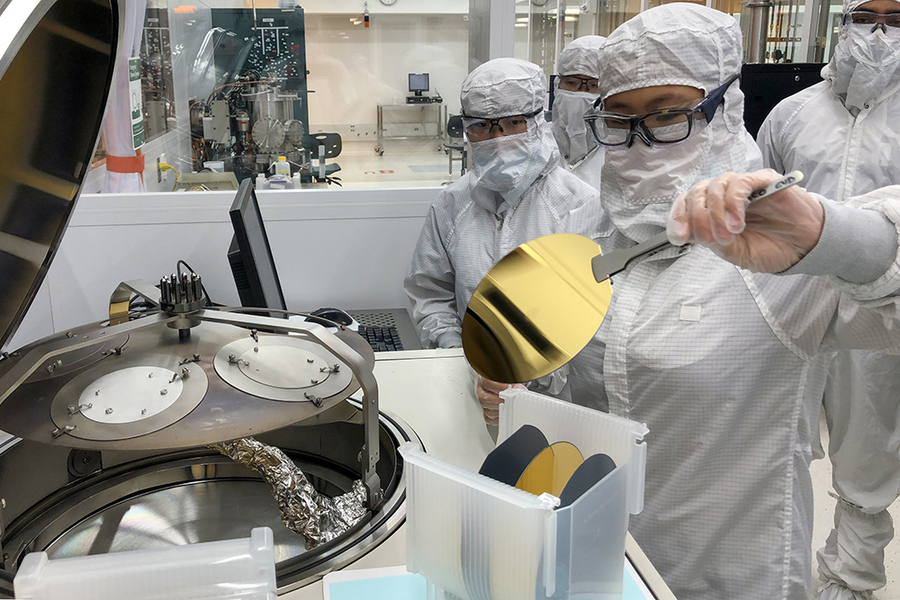The photograph depicts an indoor scene within a highly technical and clean laboratory or manufacturing facility. The setting suggests a controlled environment, potentially for handling sensitive materials. On the right side of the image, four individuals are fully donned in white cleanroom suits designed to prevent any contamination; these suits cover their entire bodies, including their hair, nose, and mouth, and are complemented by protective goggles and gloves. They appear to be of Asian descent. The person closest to the foreground is delicately handling a shiny golden disc with scientific tongs, seemingly placing it into a sophisticated centrifugal machine located near the left side of the photograph. This technologically advanced piece of equipment underscores the importance of maintaining a pristine environment, as highlighted by the presence of such extensive protective gear. Through a window in the background, there is a view of an adjacent room equipped with various lab accessories, including PCs, an office desk, and an office chair, further emphasizing the complex and technical nature of this setting.